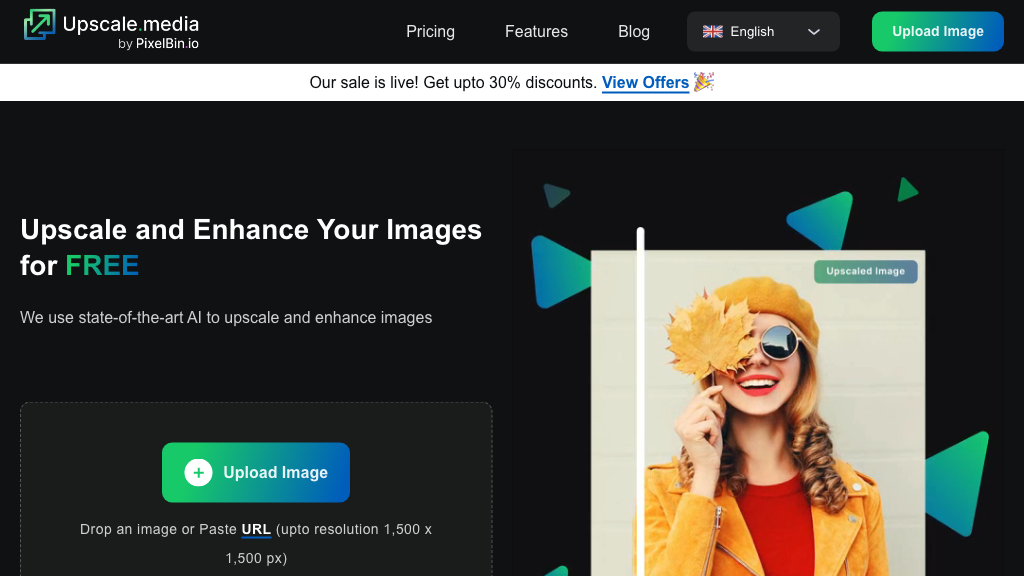**Detailed Caption:**

The landing page of our website features a streamlined, user-friendly design. On the left-hand side, there are two interlocking squares bordered in green and blue with teal accents. An arrow runs through both squares, and within them, the text reads "Upscale Media" in white, transitioning to "Buy" in grey, and then reverting to white for "Pixelbin.io".

To the right, within a black puzzle-shaped area, are buttons labeled "Pricing", "Features", and "Blog". A dark black drop-down menu displays English as the site's language. Adjacent to this, a green, teal, and dark blue button labeled "Upload Image" stands out.

Below this, a white bezel with a slight hint of grey announces "Our scale is live!" followed by an offer of "up to 30% discounts". A hyperlinked phrase, "View offers", is presented in blue text, complemented by celebratory graffiti on the right.

In a black section underneath, the text "Upscale and enhance your images for free" is displayed, with "free" highlighted in green, dark blue, and teal. Below this, a description reads "We use state of the art AI to upscale and enhance images". An off-black area features a dark grey-black square button labeled "Upload Image".

Additionally, there is a white circle with a cross, and beneath it, the instruction "Drag and drop an image or paste", followed by "URL" in bold white text with a blue underline. The parenthetical note specifies support for resolutions "up to 1500 x 1500 px".